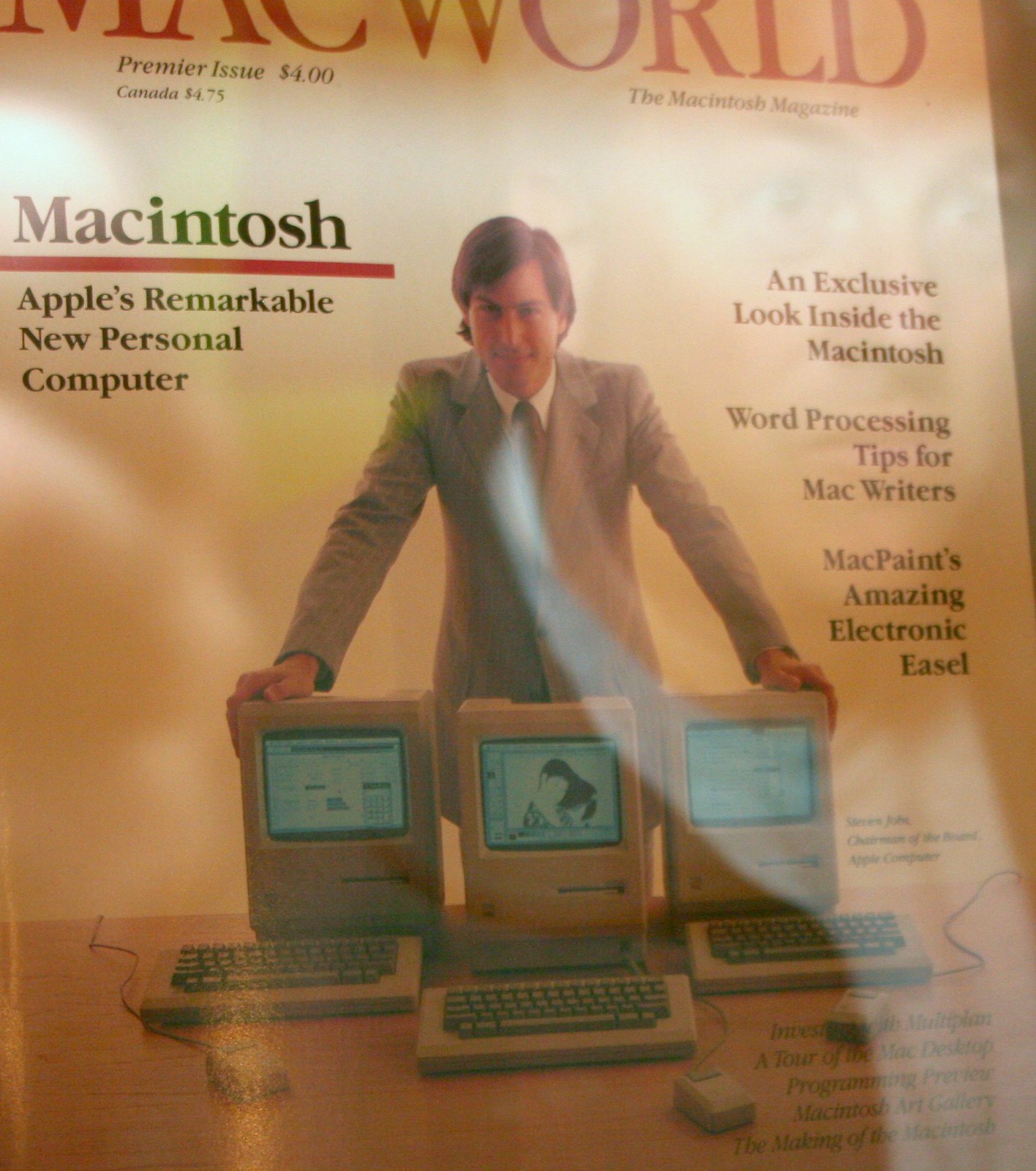The photograph captures a reflective magazine cover, specifically from Macworld's Premier Issue. The surface of the magazine is notably glossy, revealing the faint reflection of the person taking the photograph, whose face appears comically serious and startled. The primary focus of the image is a young Steve Jobs, dressed in a gray pinstripe suit, with a white shirt and tie, his medium-length hair neatly parted on the left. He is intently looking towards the camera while leaning over three early Macintosh computers, known for their tall, blocky design and 4x3 screens. Each computer is accompanied by thick, brick-like keyboards and mice. The Macworld masthead in bold red is partly visible at the top left, reading "Macworld," with “Premier Issue, $4, Canada, $4.75” printed below. Prominent text on the left announces “Macintosh, Apple’s remarkable new personal computer,” with additional headlines on the right detailing articles: “An Exclusive Look Inside the Macintosh,” “Word Processing Tips for Mac Writers,” and “Mac Paints Amazing Electronic Easel.”